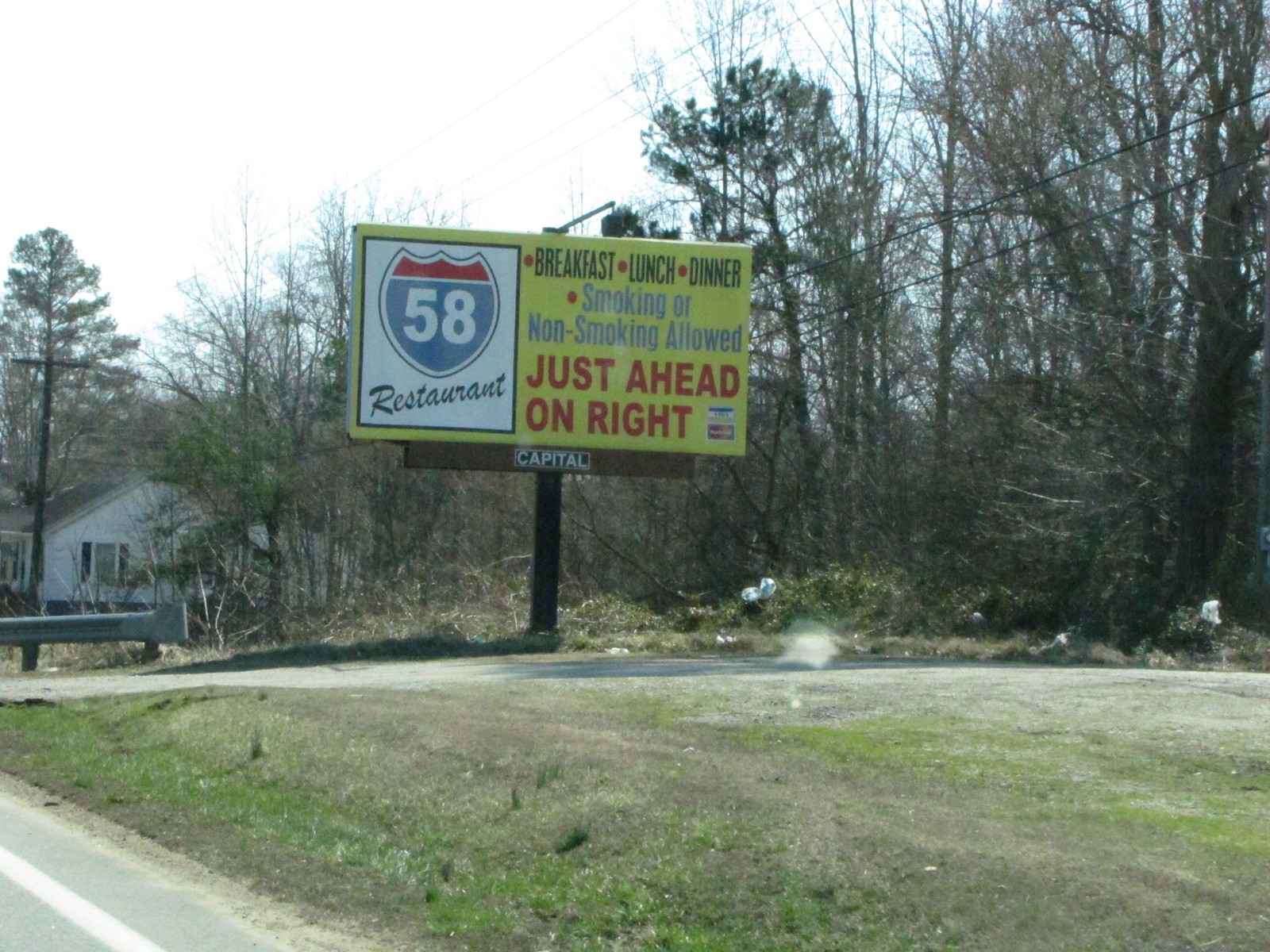The photograph depicts a grassy field with a well-maintained short lawn, interspersed with a dirt path suggesting the grass hasn't fully grown in some areas. A light gray asphalt road with a white stripe is visible at the bottom left corner. A metallic gray guardrail lines the left side of the image. In the backdrop, the right side features a tree line with power lines running across, connected to a brown pole, while the left side shows a partially obscured white house with black shutters, nestled among trees. The sky above is white, and the far background and middle ground show dead brown trees mixed with some green and brown grass.

Prominently in the middle of the image stands a tall, yellow billboard with a striking design. The billboard's black metal post supports the structure, featuring a brown border with the text "CAPITAL" inscribed on it. Above, a yellow section displays a Route 58 shield on the left, and the words "Restaurant" in cursive below it. The right side of the billboard boldly advertises "BREAKFAST, LUNCH, DINNER, SMOKING OR NON-SMOKING ALLOWED just ahead on the right."